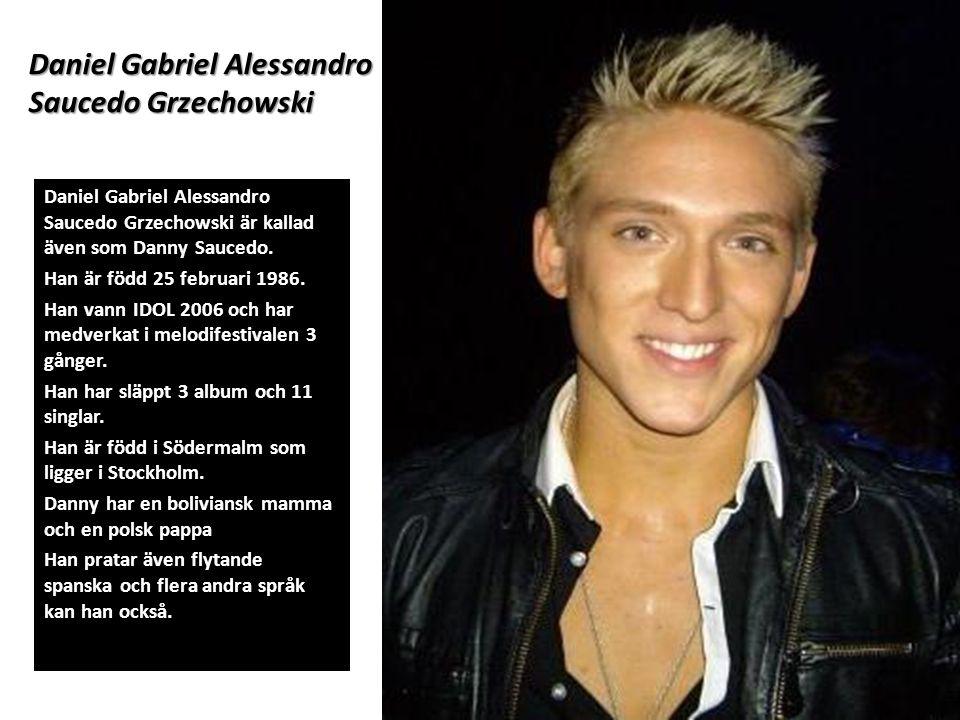In this image, we see a striking photograph of a young man named Daniel Gabriel Alessandro Saucido Zeckowski prominently positioned on the right-hand side against a stark black background. The man has blonde spiky hair, hazel eyes, and a tan complexion. He is smiling pleasantly and is dressed in a fashionable black leather jacket layered over a black and white collared shirt that buttons down the front. Around his neck, he wears a silver chain necklace partially obscured by his shirt. 

On the left side of the image, against a black box background, is a large block of text written entirely in German, potentially describing his biography or achievements. At the upper left corner, his full name, "Daniel Gabriel Alessandro Saucido Zeckowski," is prominently displayed, followed by a longer paragraph providing additional details. The overall composition and professional attire suggest that this could be an excerpt from a celebrity website or a formal presentation. The colors in the image predominantly include black, white, gray, yellow, tan, and peach, which all contribute to giving it a polished and stylized appearance.